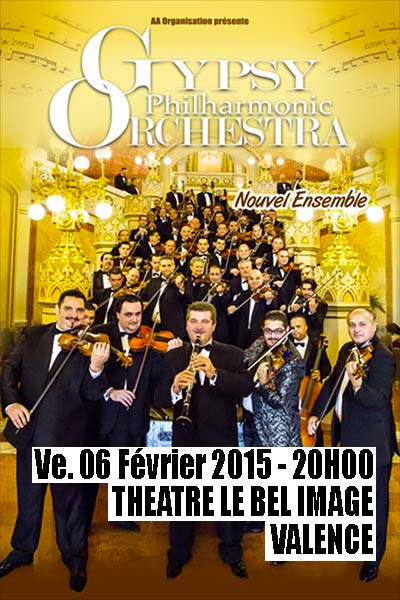This image is a vibrant and detailed advertisement poster for an orchestra performance. The background features an elegant ballroom or symphony hall lobby with a staircase filled with musicians descending in formal suits, except for one individual in a striking, garish coat. At the top of the poster, in brown text, it reads "AA Organization Presente" followed by "Gypsy Philharmonic Orchestra" in white text. Just above the stairway, in brown, is the phrase "Novel Ensemble." At the bottom, a white banner states "V.06 Fevrier 2015 - 20H00." Beneath the banner, a line in capital letters spells "THEATRE LA BELLE IMAGE." Further down, the word "Valencia" is visible, identifying the theater location. The poster's color palette includes shades of yellow, gold, brown, white, black, light blue, and dark blue, creating a visually striking composition ideal for attracting attention to the upcoming performance.